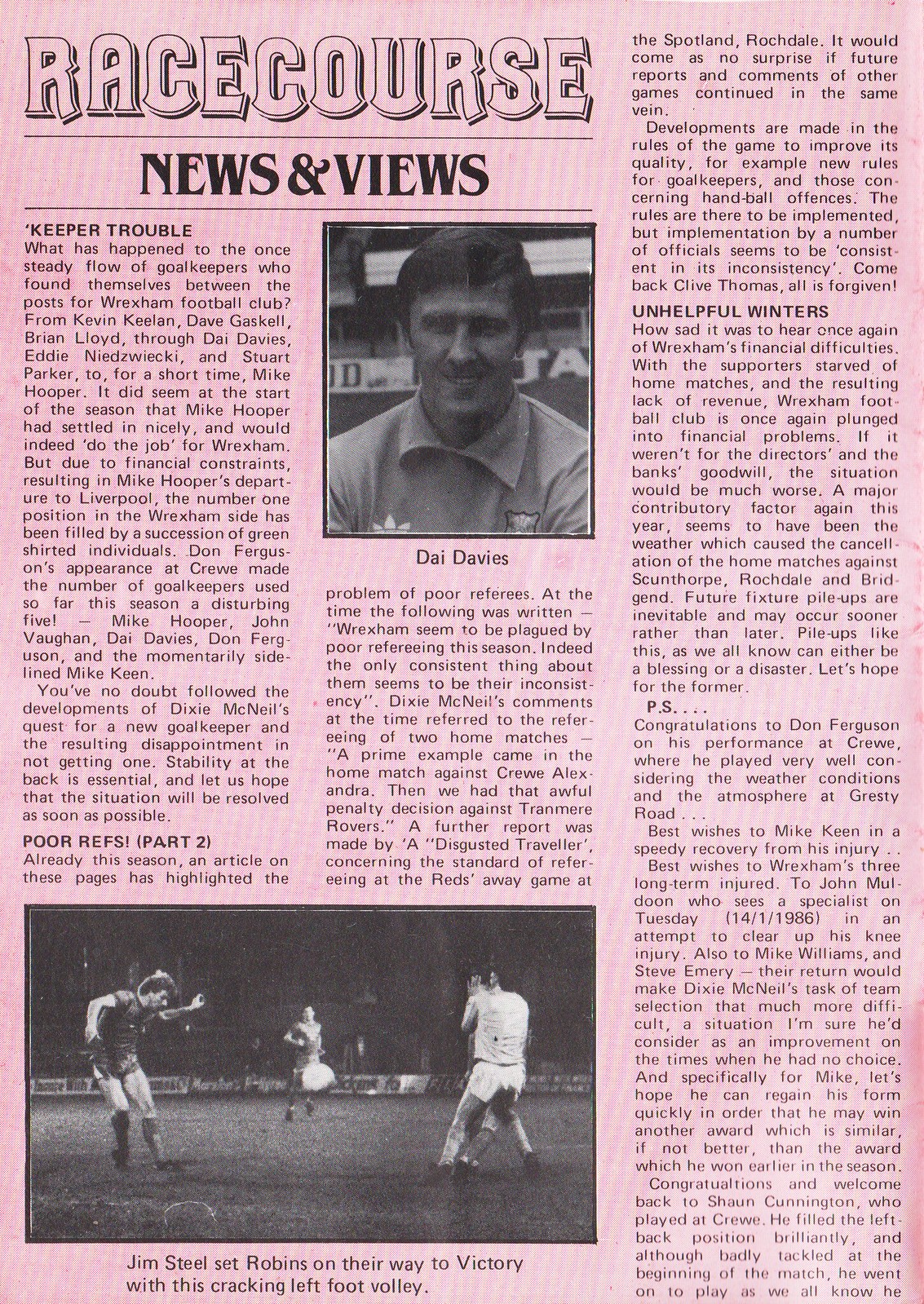The image is of a likely old, discolored newspaper page with a pinkish background that features light pink stripes. The headline at the top reads "Racecourse," followed by a subheading "News and Views." There are two black and white images on the page. The top center image depicts a man identified as "Day Davies" with accompanying text about him. The bottom left image shows players on a soccer field, with one player in a darker uniform and another in a white uniform, and underneath it is the caption, "Jim Steele set Robbins on their way to victory with this cracking left foot volley." The layout includes three short columns and one longer column on the right, filled with various articles.